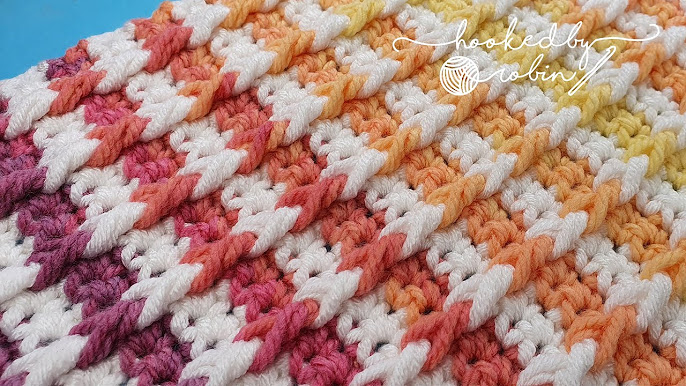The image is a photorealistic close-up of a beautifully crafted item, likely a crocheted or knitted blanket, designed by a crafter named Robin. The blanket features a captivating rainbow herringbone pattern with precise color transitions. The colors start from white at the bottom left and blend seamlessly into purple, then to pink, magenta, pale orange, and yellow, repeating this sequence throughout the design. Interspersed between these vibrant colors are distinct white stripes. A cursive inscription, "Hooked by Robin," is prominently displayed alongside a depiction of a ball of yarn and a crochet hook, signifying Robin as the creator. The overall pattern resembles a dynamic, candy cane-like strip of colors, culminating in a lively and attractive visual presentation.